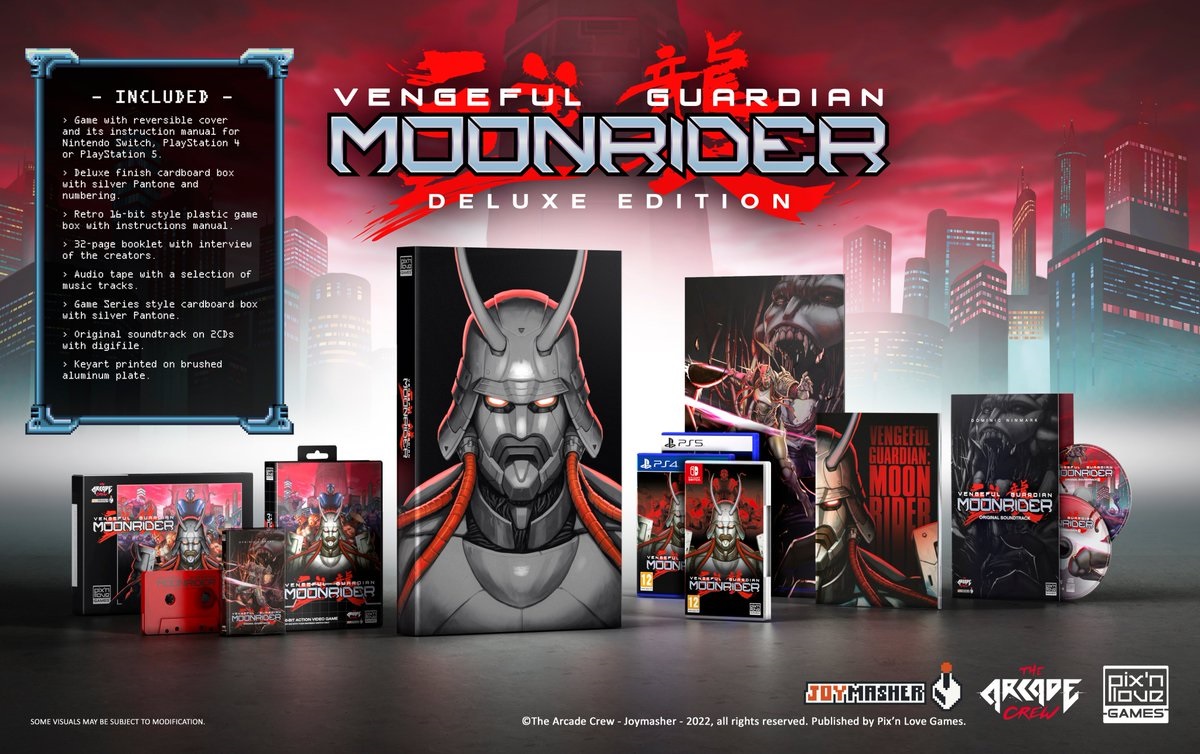This image is a rectangular advertisement for a video game titled "Vengeful Guardian Moon Rider Deluxe Edition," prominently displayed across the top. The background features a red sky and numerous lit-up skyscrapers, creating a dramatic cityscape. In the forefront, there is a detailed display of various editions of the game for different consoles, including Nintendo Switch, PlayStation 4, and PlayStation 5. Each edition has unique packaging and illustrations centered around a character wearing a helmet with two horns and red hoses that connect to what appears to be an oxygen pack.

On the left side of the image, a comprehensive list details the contents of the Deluxe Edition: a game with a reversible cover and instruction manual, a deluxe finish cardboard box with silver Pantone and numbering, a retro 16-bit style plastic game box with instructions, a 32-page booklet featuring an interview with the creators, an audiotape with selected music tracks, a series-style cardboard box with silver Pantone, the original soundtrack on two CDs with a Digifile, and key art printed on brushed aluminum plate. 

The color scheme of the advertisement is predominantly black, silver, red, and white, enhancing its striking visual appeal. The bottom right corner of the image features logos for Joy Masher, The Arcade Crew, and Pixin Love Games, confirming the collaboration behind this edition. Overall, the ad emphasizes the extensive and collectible nature of the Deluxe Edition for the game "Vengeful Guardian Moon Rider."